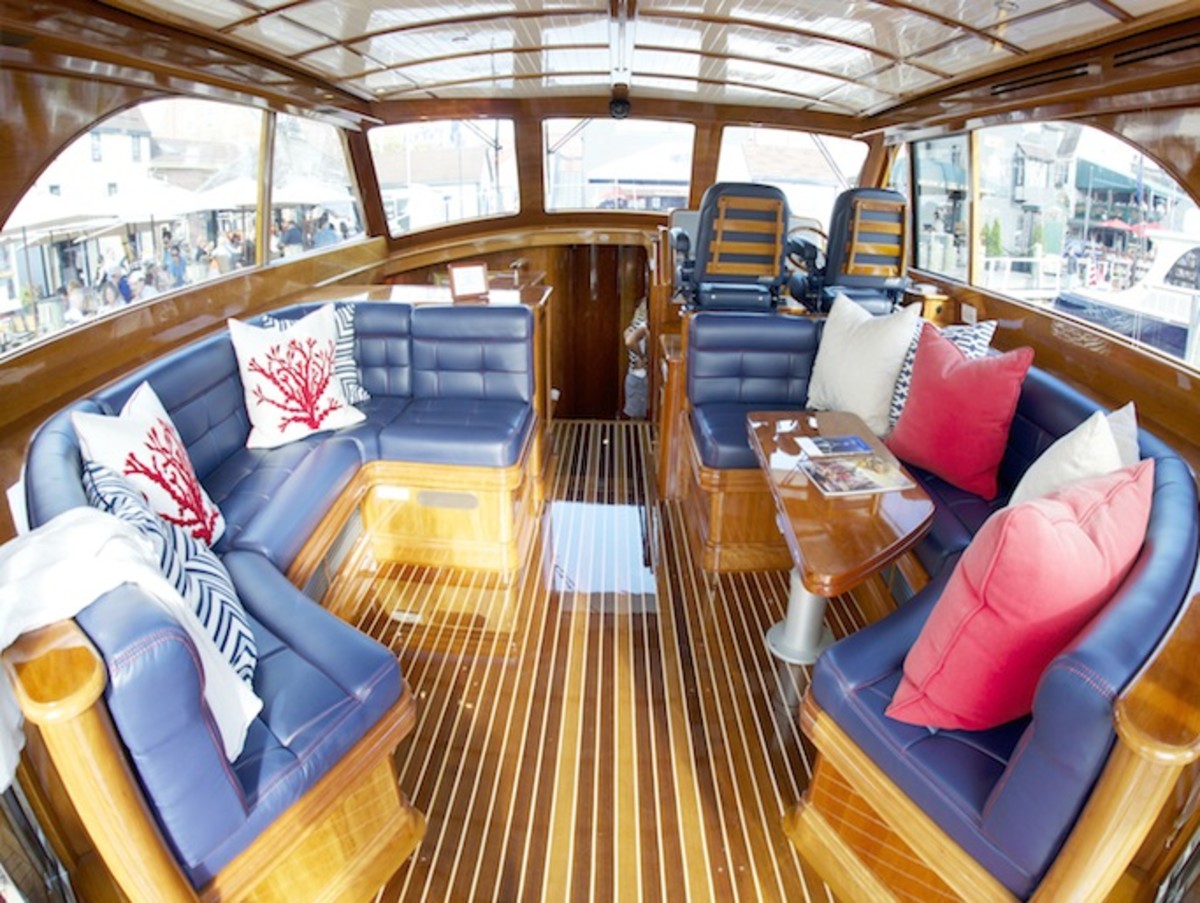The image is a color photograph depicting the interior of a traveling vessel, likely a boat given the surrounding context. The flooring is composed of beautifully polished, thin wooden slats arranged in alternating light and dark stripes. The vessel features curved seating areas crafted from light brown wood, fitted with muted blue leather cushions. The seating is adorned with an array of pillows, including red and cream-colored cushions, as well as some featuring coral designs and blue and white zigzag patterns. The benches are positioned on both sides of an aisle that leads forward and descends under the bow. There are two seats in the upper section where the steering wheel is located, indicating the control area for navigating the boat. On the right side, a wooden table with a metal base is anchored beside one of the benches, suitable for placing items like magazines. The space is framed by numerous windows wrapped in wood and topped with glass, showcasing the interior's craftsmanship. despite the elegant marine design, people can be seen outside the windows, indicating that the boat is currently on dry ground.